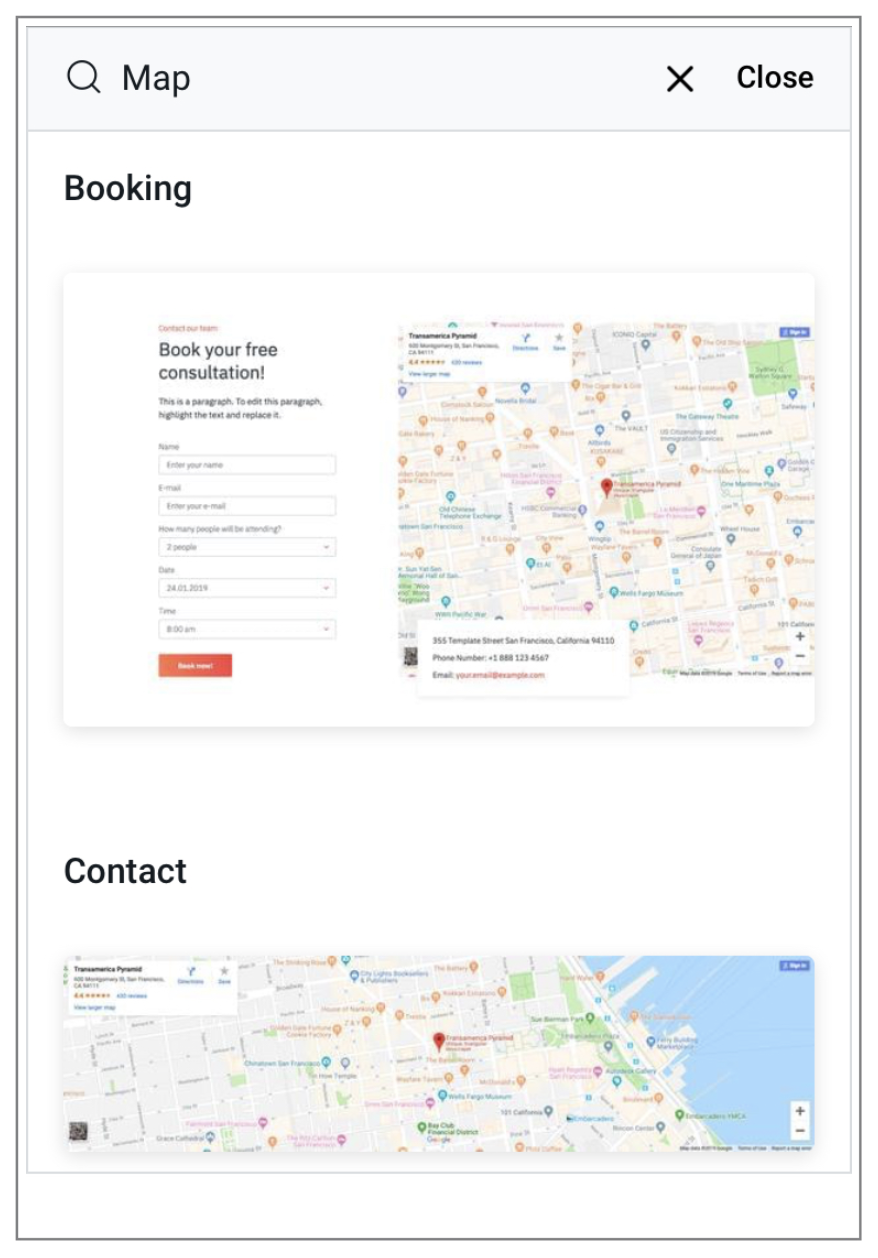In this image, there is a predominantly white background that features an interactive webpage for booking a free consultation.

- **Top Left Corner:** Displaying a portion of a map.
- **Top Right Corner:** Contains options to close the map and book your consultation.
- **Central Section:** Contains a paragraph with editable text instructions:
  - *To edit this paragraph, highlight the text and replace it*.
  - Fields for user input:
    - *Name*: Enter your name.
    - *Email*: Enter your email.
    - *How many people will be attending*: Example entry of two people.
    - *Date*: Example entry of 24-01-2019.
    - *Time*: Example entry of 8 a.m.
  - A "Book Now" button.
  
- **Bottom Section:**
  - Contact Information:
    - *Location*: Transamerica Pyramid in San Francisco, California.
    - *Rated*: 4.4 stars.
    - *ZIP Code*: 94110.
  - Additional map displaying themed locations such as restaurants, with a pinned location at the center marking the Transamerica Pyramid.
  - A phone number for further inquiries: +1-888-123-4567.

The organized and detailed layout facilitates easy navigation and interaction for booking consultations.